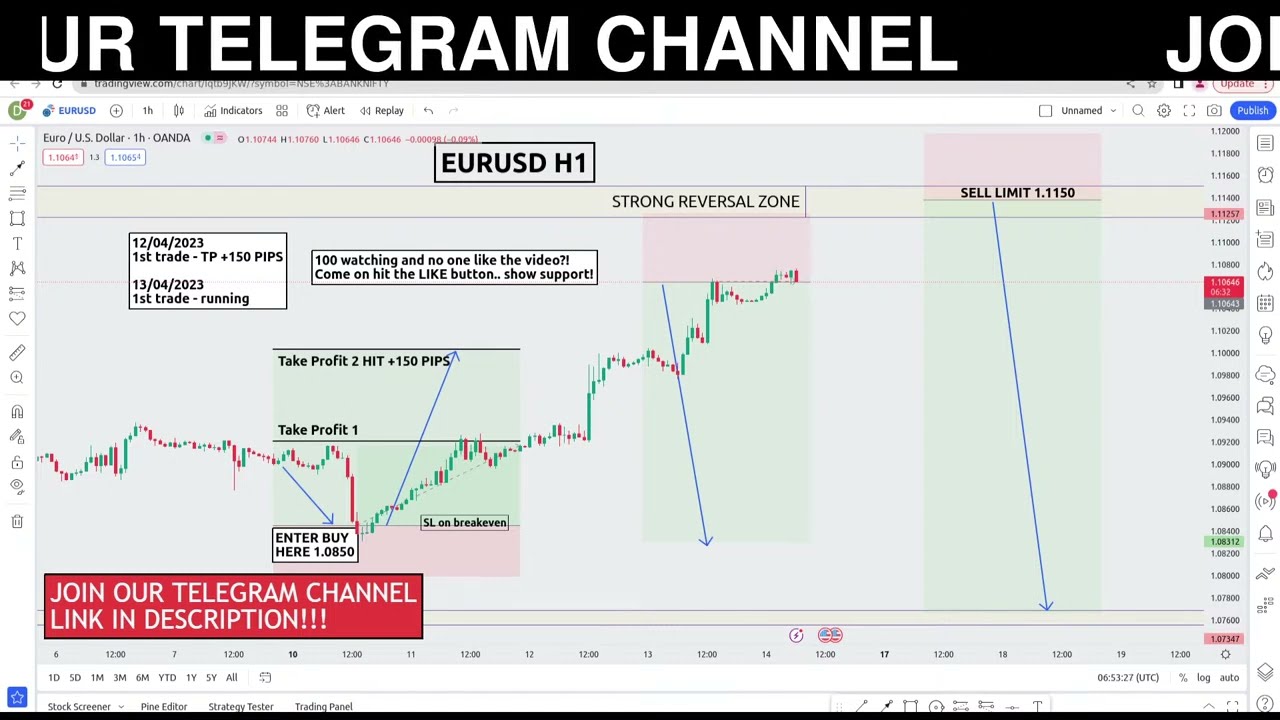This image is a detailed screenshot from a computer or device, likely showcasing a trading report relevant to currency or stock market analysis. At the top, there's a black bar featuring "UR Telegram Channel" in white font, with a partial "J0" visible on the right. Below this bar, and dominating the screen, is a complex trading graph labeled "EURUSD H1" inside a black-outlined box. Between the telegram channel label and the graph, various terms such as "alert" and "EURUSD" appear, alongside numerous icons and numbers positioned vertically on both sides of the screen.

The graph itself displays fluctuating data points with lines and annotations, including references to "first trade TP plus 150 PIPS" dated "12-04-2023" and "first trade running" dated "13-04-2023". In the middle of the screen, there is a section denoted as "strong reversal zone," along with other trading terms like "take profit hits," "TP1 and TP2," and "sell limit 1.1150." Additional details include SL (Stop Loss) and a plotted path showing different price movements.

The lower-left corner prominently features an advertisement text "Join our Telegram channel, link in description," suggesting this image serves both as an analytical tool and a promotional piece. Overall, the screenshot includes detailed trading data, relevant alerts, trading strategy points, and a call to action for engaging with the Telegram channel.